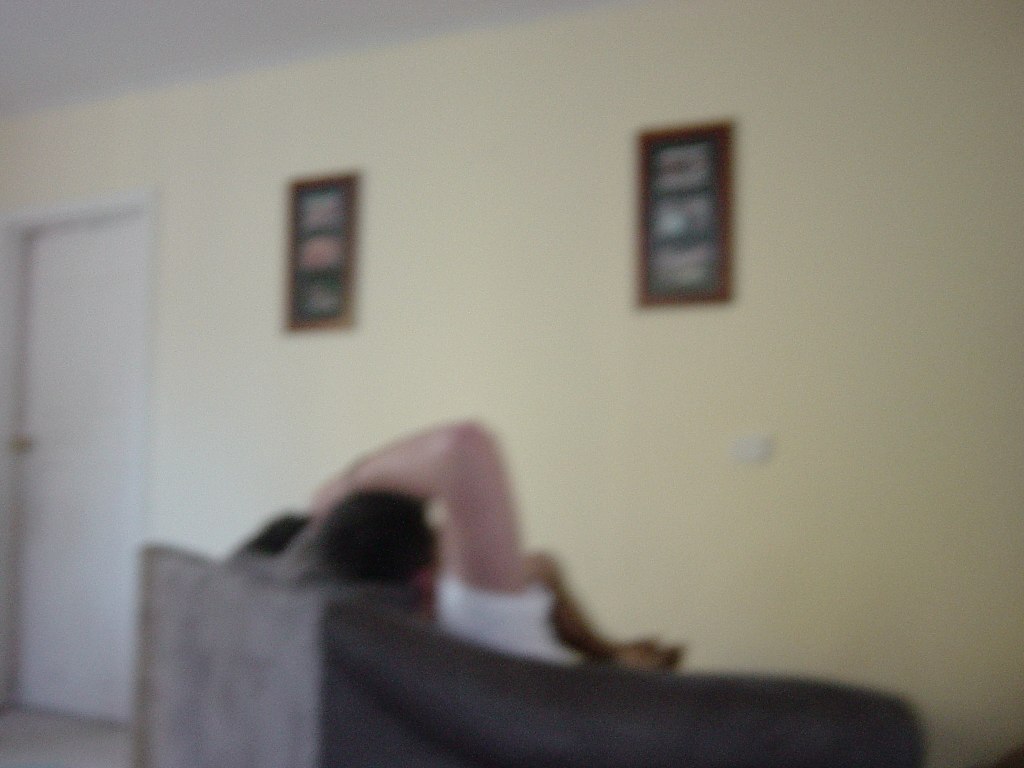This indoor image, slightly grainy and out of focus, prominently features a yellow wall that occupies the majority of the composition. In the top right corner, a white ceiling is visible, while a closed white door lines the left edge of the photograph. Adorning the wall are two rectangular picture frames made of brown wood, each holding three separate images. Near the bottom of the picture is a piece of furniture, possibly a chair or couch, facing the wall. Seated on this furniture is a person with light skin, whose gender is indistinguishable. They are clad in a white short-sleeved shirt and have dark hair. Their right arm is bent at the elbow with their hand resting on their head.